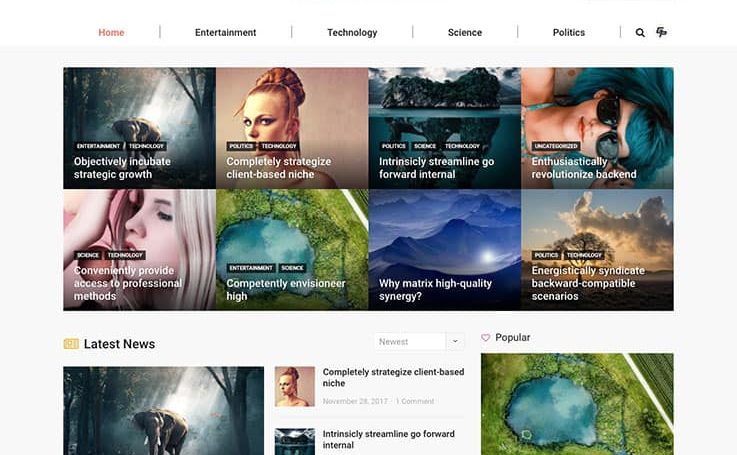**Website Screenshot Description**

At the top of the screenshot, there is a navigation bar featuring category labels. The current category, highlighted in an orangish-red color, is "Home". Adjacent categories, displayed in black, include "Entertainment," "Technology," "Science," and "Politics." To the right, there is an eyeglass icon symbolizing a search function, and an adjacent icon labeled "CP."

Below the navigation bar, eight square banners are arranged in two rows, each with unique images and captions:

1. **Image of an Elephant in a Woodland:** The caption reads, "Objectively Incubate Strategic Growth."
2. **Woman with Hair in a Bun:** The caption reads, "Completely Strategize Client-Based Niche."
3. **Mountain Range with a Lake or Pond:** The caption reads, "Intrinsically Streamline Go-Forward Internal."
4. **Woman with Sunglasses and Blue Hair:** The caption reads, "Enthusiastically Revolutionize Backend."

Starting the next row:

5. **Woman Holding an Object to Her Face (Unclear):** The caption reads, "Conveniently Provide Access to Professional Methods."
6. **Aerial View of Greenery Surrounding a Pond or Lake:** The caption reads, "Competently Envisioneer High."
7. **Night Sky Over Mountain Range with a Bright Light:** The caption reads, "Why Matrix High Quality Synergy."
8. **Lone Tree with a Background of Clouds and Sun (Sunrise or Sunset):** The caption reads, "Energistically Syndicate Backward Compatible Scenarios."

Below the banners, there is a section labeled "Latest News," featuring a few icons similar to those in the navigation bar, though the specific details are not entirely legible.